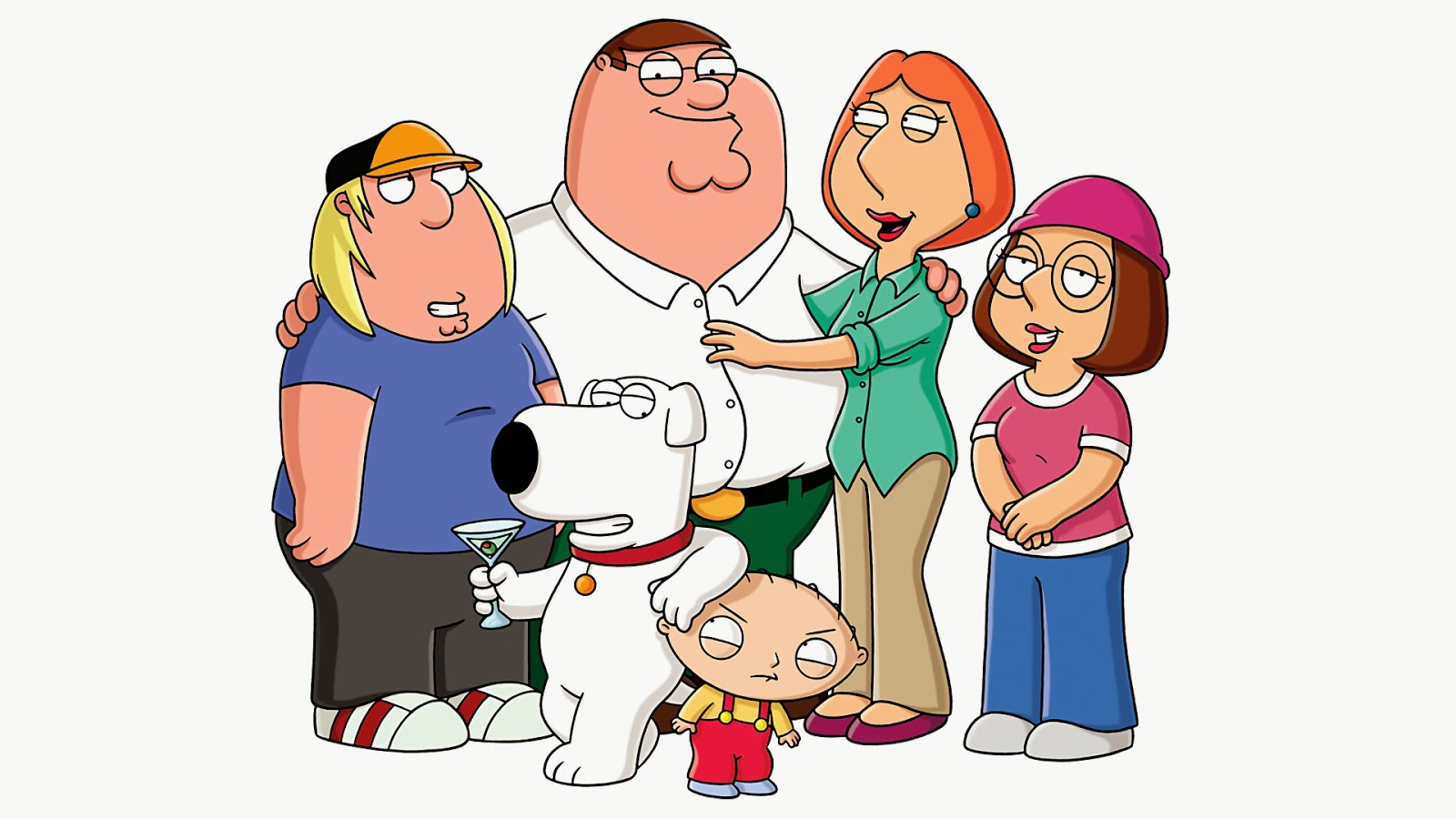This image showcases the Griffin family from the TV show Family Guy, created by Seth MacFarlane. The scene is set against a very light gray or off-white background, framed in a horizontal rectangle. In the center stands the large, bespectacled Peter Griffin, sporting a white collared shirt, green pants, a black belt with a gold oval buckle. To Peter's right is his wife, Lois, dressed in a green button-up collared shirt, untucked over her khaki pants, and purple loafers. She is looking at Peter warmly. 

To Peter's left is their teenage son, Chris Griffin, identifiable by his long blonde hair underneath a black and orange baseball cap. He is wearing a blue short-sleeved t-shirt, gray pants, and white and red sneakers, looking towards his father. On the far right stands their daughter, Meg Griffin, in a pink beanie cap and large glasses. She is dressed in a matching pink t-shirt with white trim, blue pants, and gray shoes.

At the forefront of the image are the youngest members of the family. Stewie, the baby, stands with an oval-shaped head, wearing red overalls over a yellow long-sleeved shirt and gray shoes. He looks annoyed as the family's anthropomorphic white dog, Brian, leans on him. Brian, donning a red collar, stands upright holding a martini glass with an olive, his paw resting on Stewie's shoulder. 

The entire family is gathered closely, with everyone except Stewie smiling, showcasing their typical family dynamic in the style of the beloved animated series. As is often depicted in the show, Meg stands somewhat apart from the family, with Peter hugging Lois and Chris but not her. This image captures the essence of the Griffin family in their regular outfits and positions them true to their character traits.